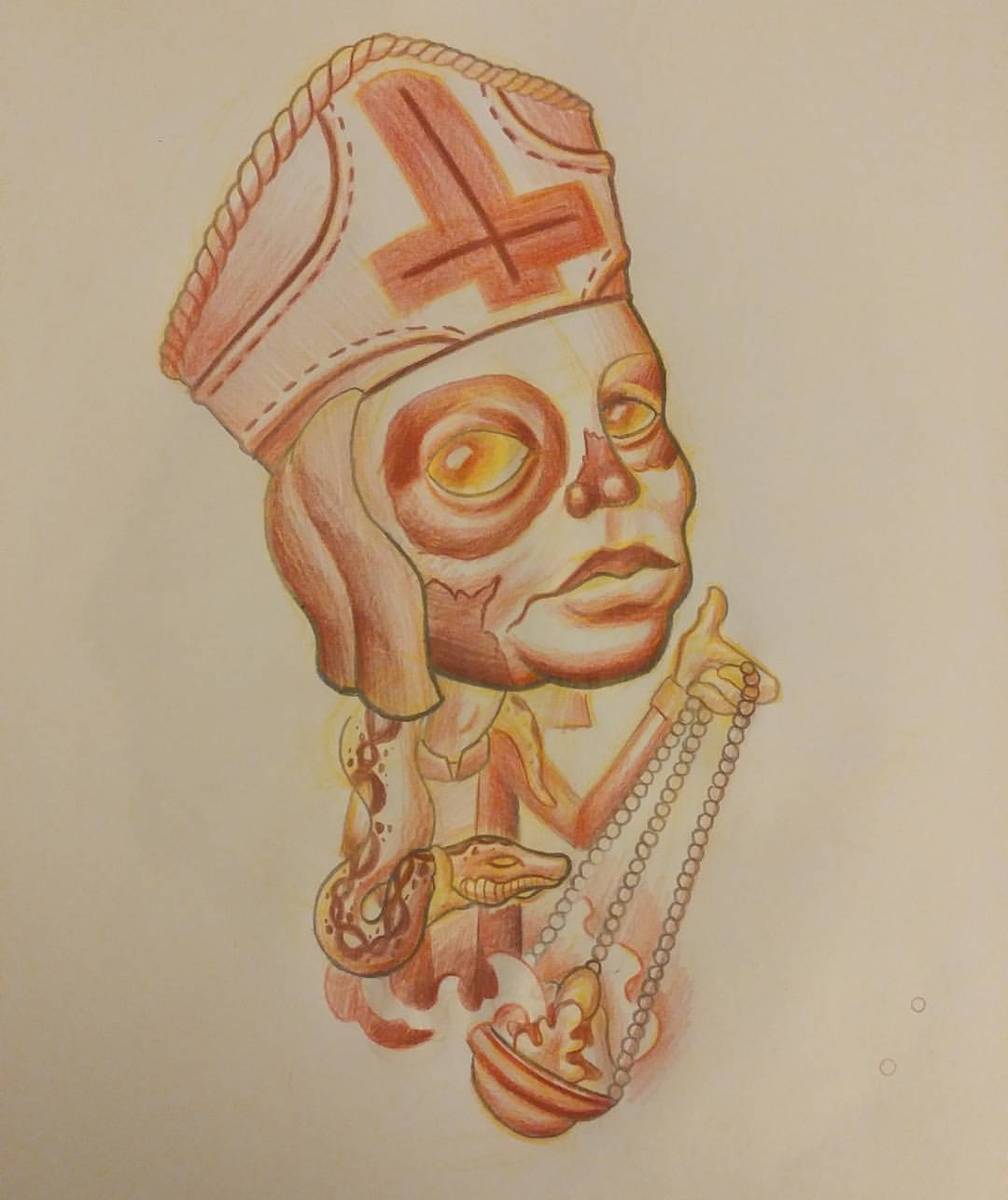This detailed and vivid drawing, rendered on tan paper with orange, yellow, and white tones, depicts a menacing, possibly satanic religious figure. The figure's face, which is charred and partially rotting, features dark brown circles around large impassive yellow eyes. An upside-down cross adorns a tall hat reminiscent of a bishop’s mitre, marking the figure's sinister nature. A tan and yellow snake coils around the figure’s small body and neck, adding to the eerie aura. The figure is attired in a white shirt and black jacket, with a scarf draped over the back of the neck and head, and a rope-like piece encircling the top of the head. In one hand, the figure holds a beaded censer or chalice, swinging it to release visible tendrils of smoke, enhancing the otherworldly atmosphere. The reddish-brown and burnt yellow hues contribute to the drawing’s overall dark, unsettling theme.